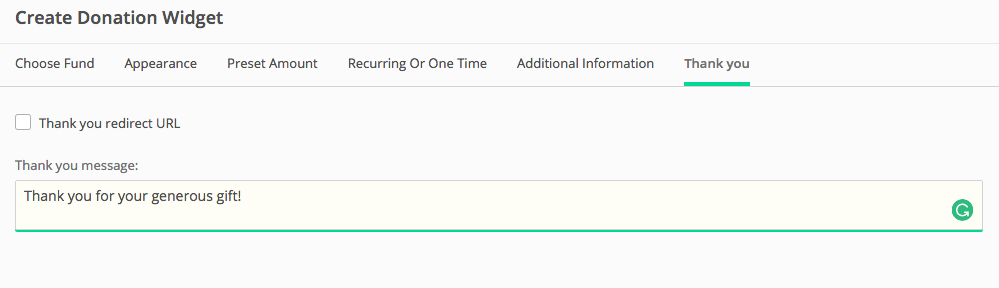"Create a donation widget featuring several customization options. Users can select from various funds and adjust the widget's appearance. They can also choose preset donation amounts, and specify whether the donation is recurring or a one-time contribution. Additional information fields are available. A 'Thank You' message, with an accompanying green underline, appears. There's also an optional redirect URL presented with an unchecked checkbox beside it, followed by another 'Thank You' message that reads: 'Thank you for your generous gift!' A green refresh button is located to the far right of this message, followed by another green underline beneath the text field."